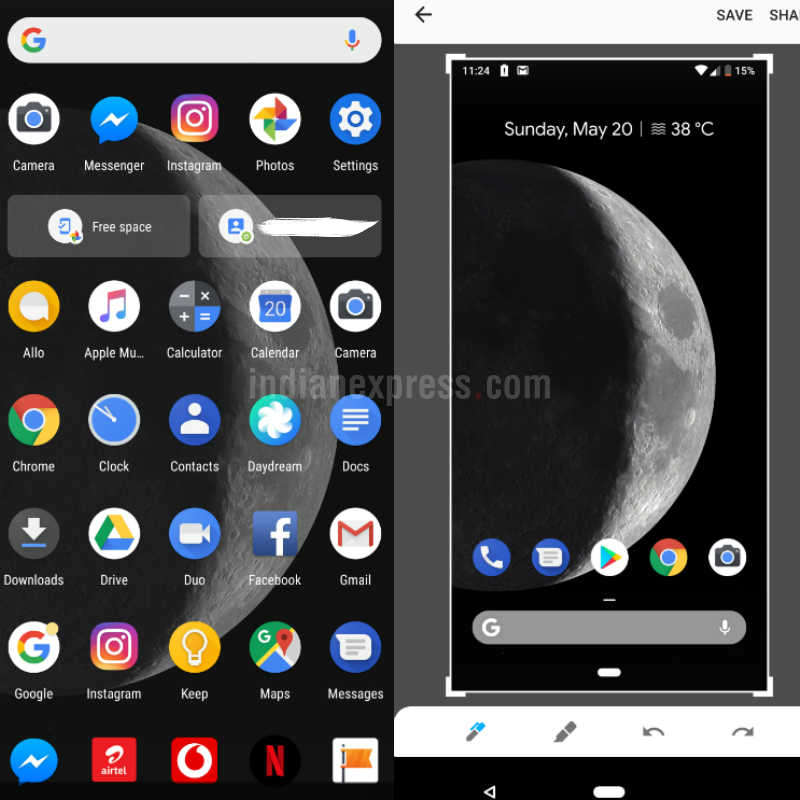This vertical image, styled for a smartphone device, gives an impression of two distinct sections divided down the middle. On the left side, the background is a deep black, featuring a depiction of the moon. The moon appears in lighter gray, with its left side shadowed and its right side illuminated. 

At the top of the screen is a Google Search bar with a microphone icon, followed by an array of app icons with their respective labels, including Camera, Messenger, Instagram, Photos, and Settings. The list continues with various apps: Allo, Apple Music, Calculator, Calendar, Camera, Chrome, Clock, Contacts, Daydream, Docs, Downloads, Drive, Duo, Facebook, Gmail, Google, Instagram, Keep, Maps, Messages, and Netflix.

The lower portion features a navigation bar with an arrow for going back, and save and share options on the top right. This section has a medium gray background and showcases the date, Sunday, May 20th, alongside the temperature at 38 degrees Celsius. The icons for battery life, time, and the moon reappear here, maintaining a cohesive visual theme. Finally, at the bottom, several icons are present, continuing the orderly layout of the interface.